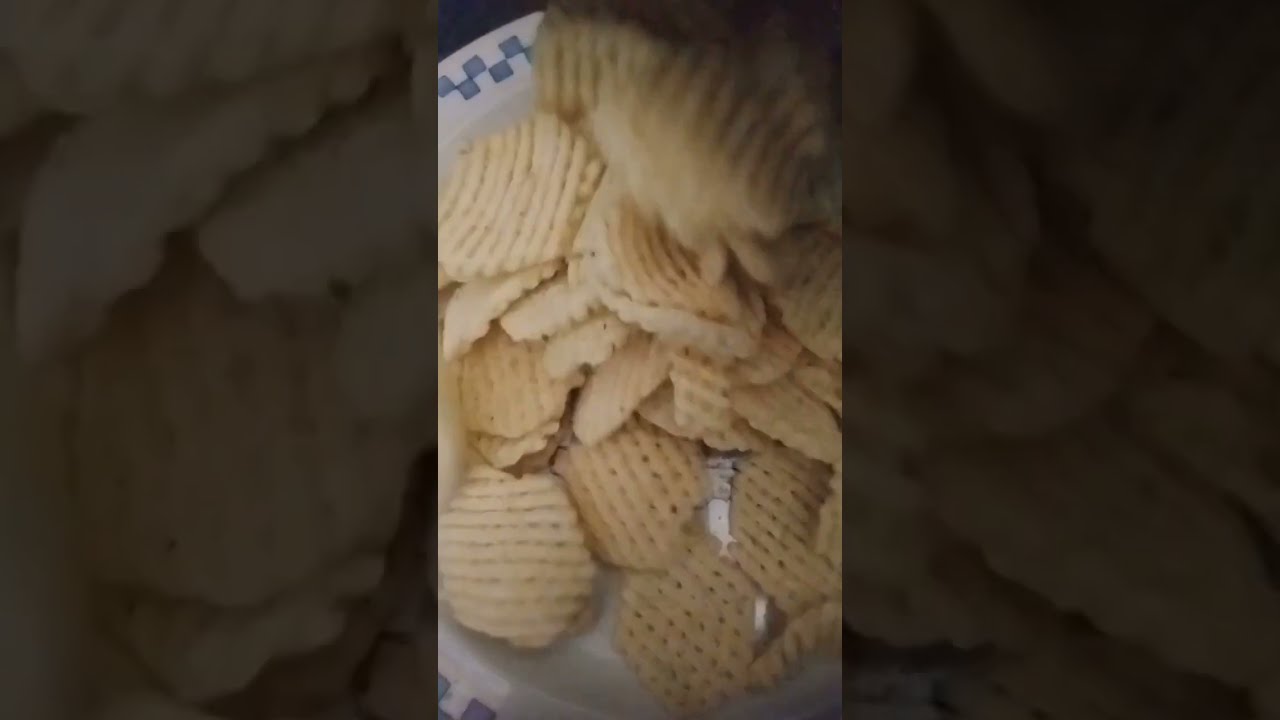The image features a close-up of a white plate with a blue checkered pattern along its rim. Positioned centrally, the plate is catching a cascade of light golden yellow, waffle-shaped potato chips, which have a distinctive crisscross pattern and flat, almost octagonal edges. These chips are being poured onto the plate, suggesting they are either freshly served or falling from a container. The image composition is divided into thirds: the center section, in sharp focus, vividly highlights the plate and the falling chips. In contrast, the left and right thirds of the image are grayed out and blurred, presenting enlarged, less distinct replications of the central image, emphasizing the focus on the detailed scene in the center. The background is also a grayed-out, zoomed-in version of the central image, further reinforcing the visual emphasis on the crisp, intricately patterned chips against the elegantly bordered plate. The scene appears to be set indoors.